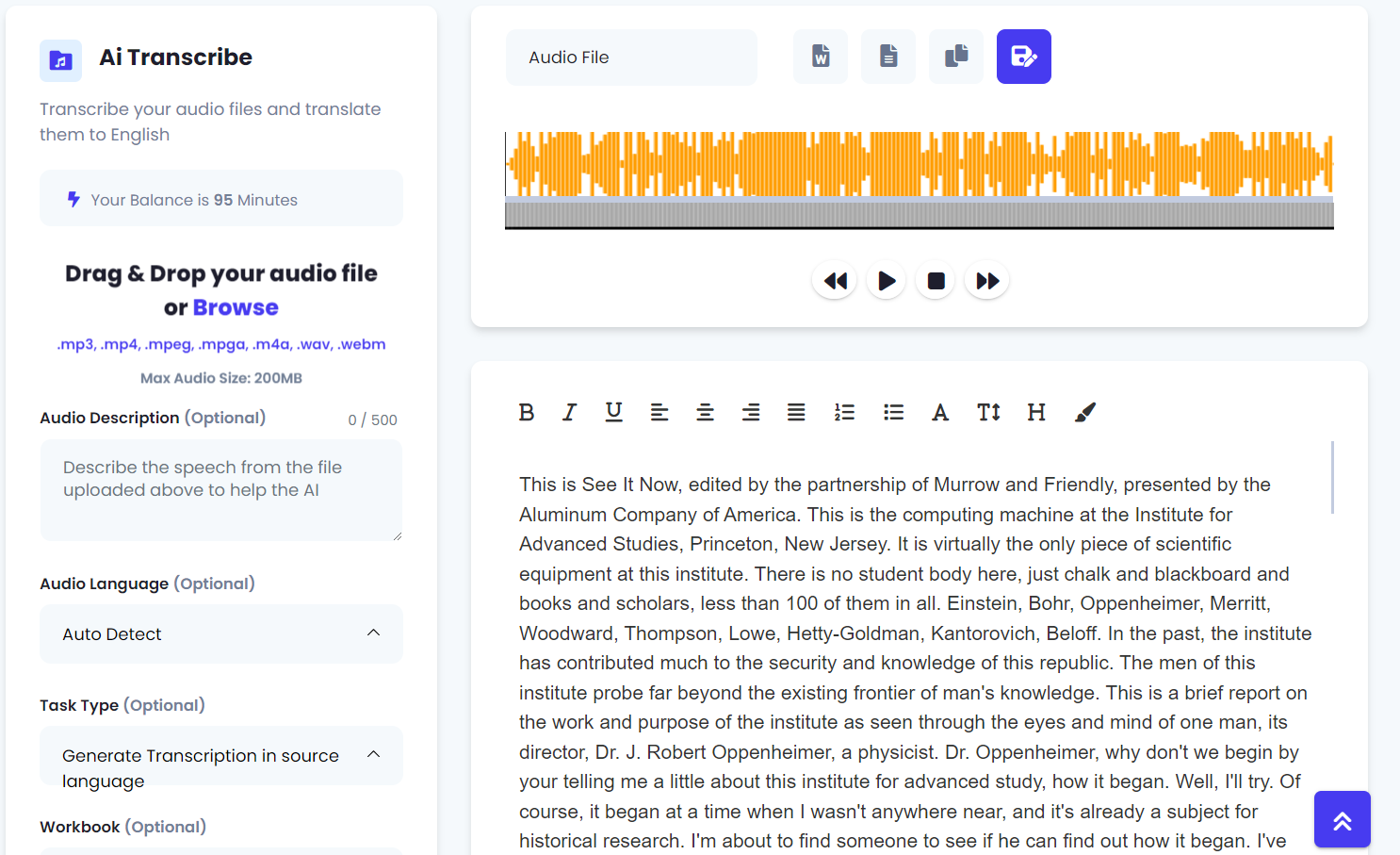Here's a more detailed and descriptive caption for the photo:

---

The image displays the user interface of a transcription and translation software. On the left side of the screen, there is a text input box where users can type in various prompts or commands. To the right, there's a preview area that shows the output of the text being entered. At the top of this section, a header prominently reads “AI Transcribe,” followed by the subtext, “Transcribe your audio files and translate them to English.” It also displays the user's available balance of transcription minutes, which is currently at 95 minutes.

Below this, there is a specific audio description feature selected, described as “Describe the speech from the file uploaded above to help the AI.” Various options for customization are presented, allowing users to format the transcribed text with bold, italic, or underline styles, similar to editing capabilities in word processing software.

Above the main working area, there is an additional section that visualizes real-time voice waves as the audio is being recorded and transcribed. This section includes playback controls, allowing users to pause, play, rewind, or fast-forward through the audio file.